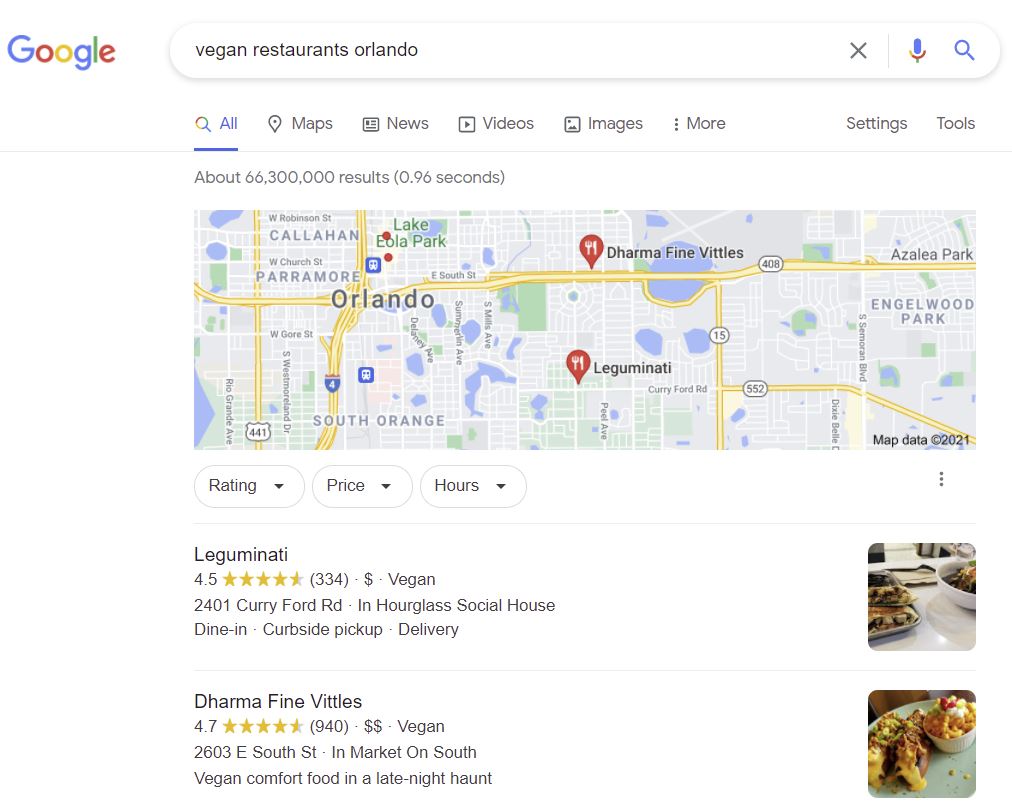Screenshot of a computer screen displaying a Google search for "vegan restaurants Orlando." The upper left corner features the colorful Google logo comprised of blue, red, yellow, and green letters. Below the logo, a search bar contains the typed query "vegan restaurants Orlando," flanked by an 'X,' a microphone icon, and a search button.

Under the search bar, a navigation row offers options: All, Maps, News, Videos, Images, More, Settings, and Tools. The central part of the screen shows a colorful map of Orlando, highlighting major highways in yellow and smaller streets in white. Two locations are pinned on the map: Dharma Fine Vittles and Lake Uminati.

Below the map, an interactive button allows users to filter search results by rating, price, and hours. The first listing is for Lake Uminati, rated 4.5 stars with three dollar signs indicating its price range. This vegan restaurant, located at 2401 Curry Ford Road within the Hourglass Social House, offers dine-in, curbside pickup, and delivery options. A corresponding image showcases a bowl of food alongside a tray.

The next listing features Dharma Fine Vittles, boasting a 4.7-star rating and two dollar signs for its price range. Situated at 2603 East South Street in Market on South, this venue is known for vegan comfort food and as a late-night haunt. Accompanying the description is a photo of sauced vegan dishes, including a brown-colored main course topped with orange sauce and a small condiment bowl with a grape garnish.